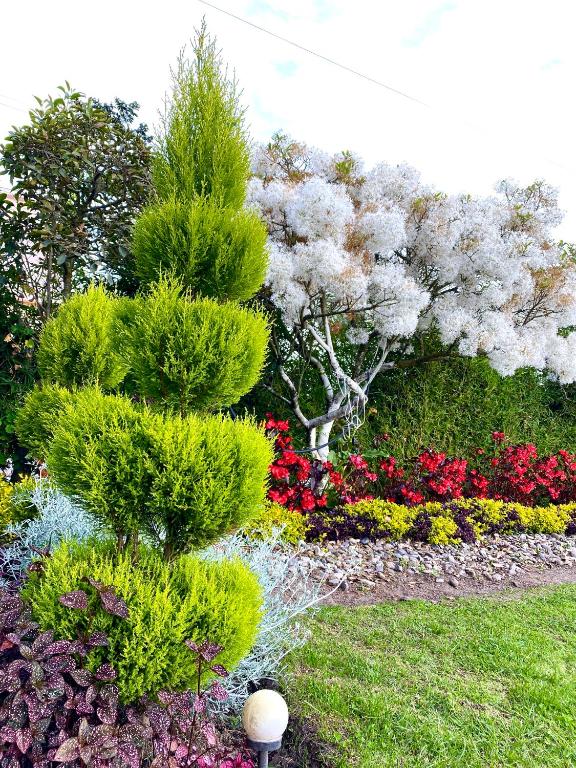The image captures a well-manicured garden on a mostly cloudy yet pleasant day. The foreground features a meticulously maintained grassy area, and towards the bottom right, there's a light fixture with a round bulb. On the left side of the image, a distinctive tree or bush has been trimmed into five stacked circular layers. The garden showcases various foliage and vibrant rows of flowers: pinkish flowers at the base, followed by red and yellow blooms. A visually striking tree with white bark and white leaves stands out against a backdrop of green trees and bushes. The scene is complemented by a row of rocks and some dirt just above the grass. Intriguingly, a gray line runs diagonally across the sky from the top left to the bottom right, possibly an artifact but adding an enigmatic element to the photo. Overall, the image portrays an exquisite and thoughtfully arranged garden landscape.